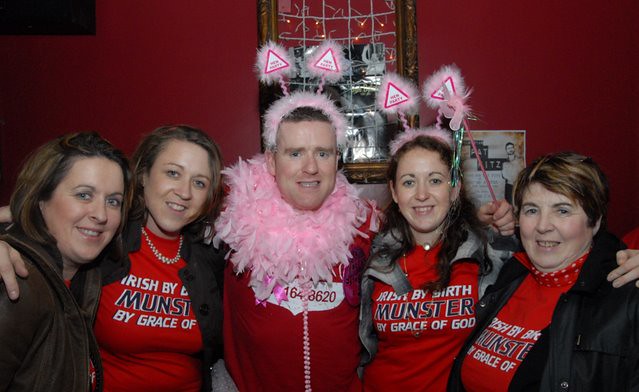The image depicts a group of five people, all wearing matching red shirts that read, "Irish by birth, Munster, grace of God." Central to the group is a man in his 30s, adorned with a pink feather boa and a leather headband featuring two fluffy pink triangle ears. To his right stands a cheerful woman in her late 20s or early 30s with long brown hair, also sporting a matching headband and holding a pink wand that he’s gripping around her shoulders. To her right is an older woman, likely in her early 50s, smiling while wearing a black jacket over her shirt. On the left of the man is another woman with shoulder-length brown hair, wearing a silver necklace and a black jacket. Finally, completing the group on the far left, is a woman with medium brown hair and a black jacket over her red shirt. All five are smiling with their arms around each other, set against a red backdrop, suggesting a close-knit or celebratory gathering, possibly a religious or community event.